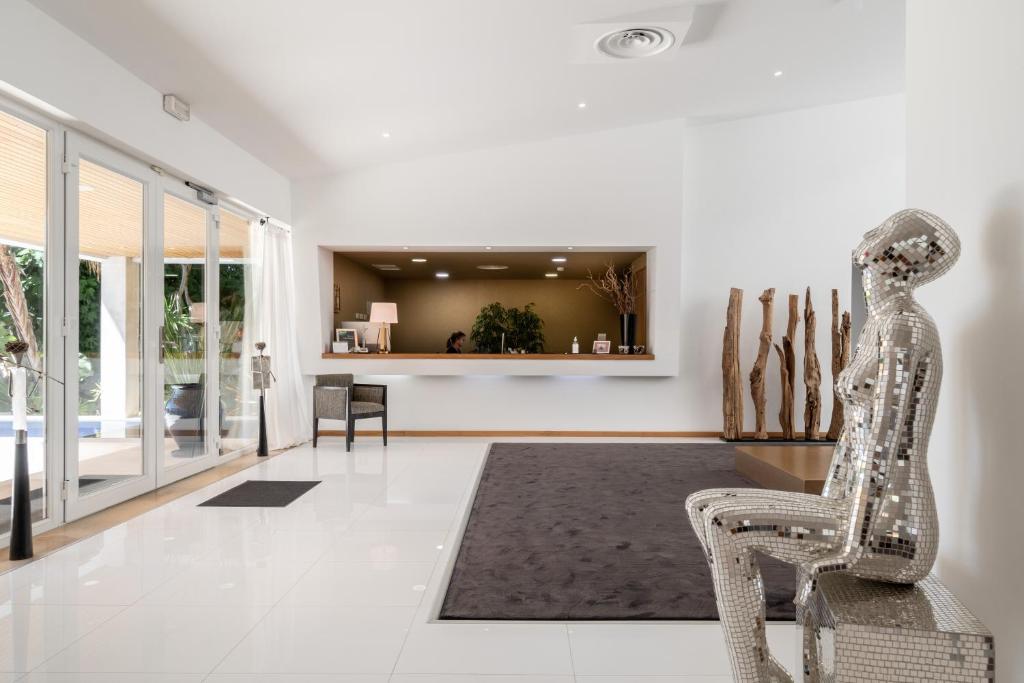This image captures the striking minimalist and industrial design of the lobby in Villa Valverde Design Country Hotel, located at the southern tip of Portugal in Lagos. The white-tiled floor reflects the abundance of natural light streaming through the large, sliding glass doors to the left, which serve as the main entrance. Directly centered is a built-in reception desk featuring a woman seated behind it, partially visible through an opening in the wall, working beside a variety of items including a lamp, a vase, bowls, a bottle, and a photo frame. The counter also hosts a small flower pot, while behind the receptionist stands a small tree.

Adding to the artistic ambiance, a mannequin composed of mirrored glass pieces sits on a matching mirrored stool in the foreground, providing a captivating focal point. Nearby, five sculptural tree branches are mounted on a sleek black base, contributing to the artistic, almost museum-like feel of the space. The lobby includes additional seating, exemplified by a gray chair positioned near the reception and a guest chair elsewhere in the room. Recessed lighting subtly enhances the aesthetic, showcasing various sculptures and industrial elements like vent fans. A large black mat guides visitors further into the hotel's interior, where they can explore other luxurious amenities, such as the spa and winery.

The décor, with its clean lines, sparse furnishings, and thoughtful artistic touches, demonstrates a well-curated blend of functionality and elegance, creating a serene yet intriguing environment for guests.